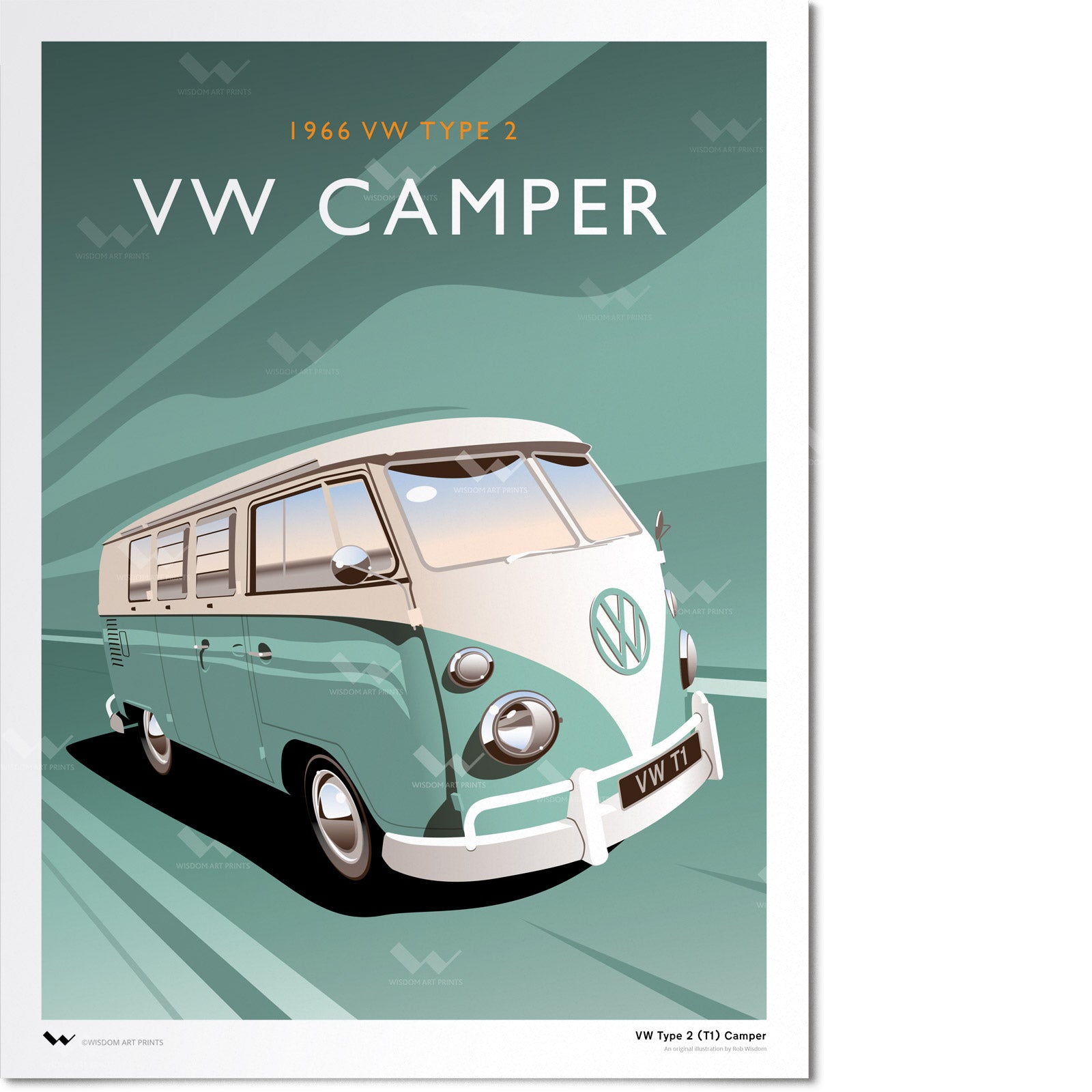This detailed color illustration appears to be either a drawing or a computer-generated image, likely used as a poster or book cover. The image features a vintage 1966 Volkswagen Type 2, commonly referred to as a "VW Camper." The titles "1966 VW Type 2" and "VW Camper" are prominently displayed at the top in large white and smaller gold letters, respectively.

The central focus is on the side profile of the iconic pillow-shaped Volkswagen bus. This van is two-toned, with the top half painted white and the bottom half a mint green or teal color. The large, circular Volkswagen logo, comprising a stylized 'V' on top of a 'W,' is notably featured on the front of the vehicle. The bus includes distinctive round headlights and rims, and it is depicted moving to the right of the frame. 

Additionally, there is a black license plate on the front of the bus that reads "VW T1." The entire image is bordered by a thick white frame, and the background shares the same teal color as the vehicle itself. The bottom left corner of the white border bears the copyright "Wisdom Art Prints," while the bottom right corner reiterates "VW Type 2 Ti Camper." A watermark with the stylized 'W' logo is scattered across the illustration, ensuring the authenticity and copyright protection of the artwork.